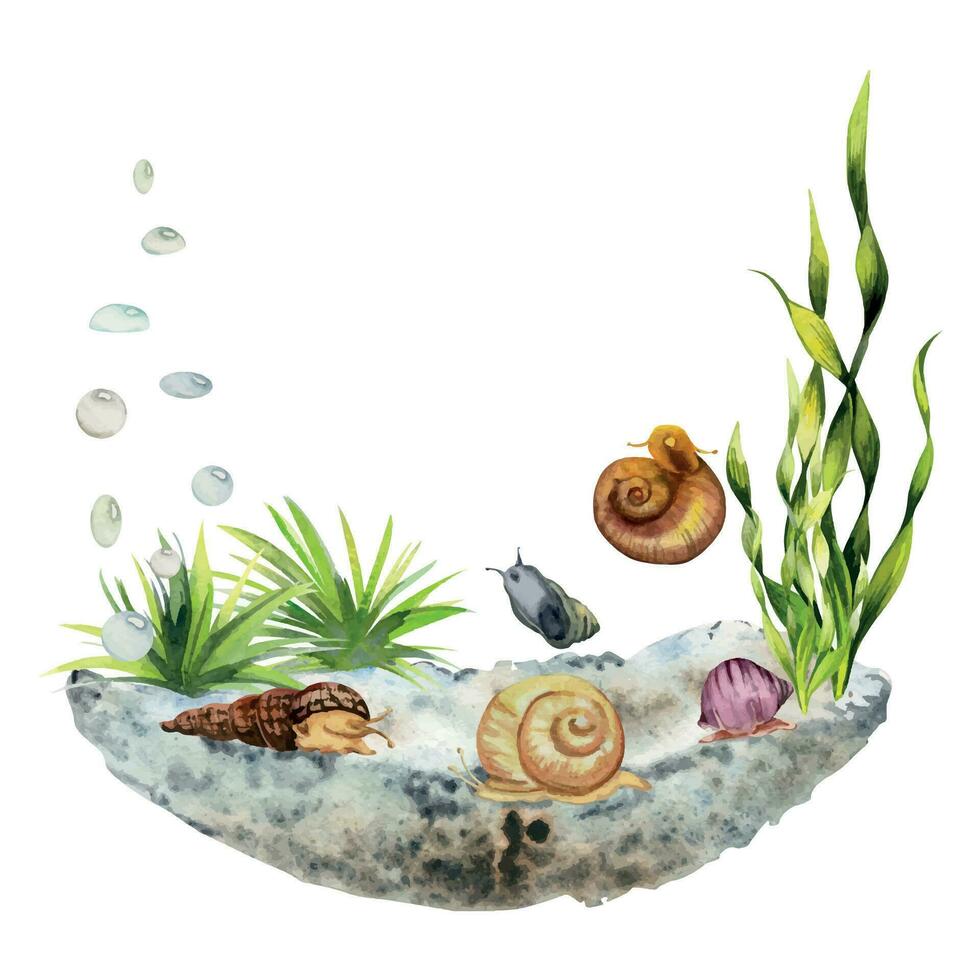This detailed watercolor illustration depicts an undersea or aquarium scene with a variety of snails inhabiting a mottled gray and black seafloor. On the right side, a tall, flowy green plant stands out, while the left side features two short, bushy, spiky-leaf plants. The snails are diverse in color and shape: In the center foreground, a light brown or tan, circular snail is prominent. To its left, a long, brown snail with a conical shell sits at the bottom. To the right of the tan snail, a lilac and dark purple snail can be found next to the green plant, which may be accompanied by a purple fish. Above the tan snail, a bluish-gray snail appears to float in the water on a white background, while another snail with a cream or orange shell is visible above the purple fish, to the left of the green plant. Additionally, a yellow and red snail adds vibrant color to the scene, and tiny blue bubbles rise up the image, enhancing the underwater ambiance.